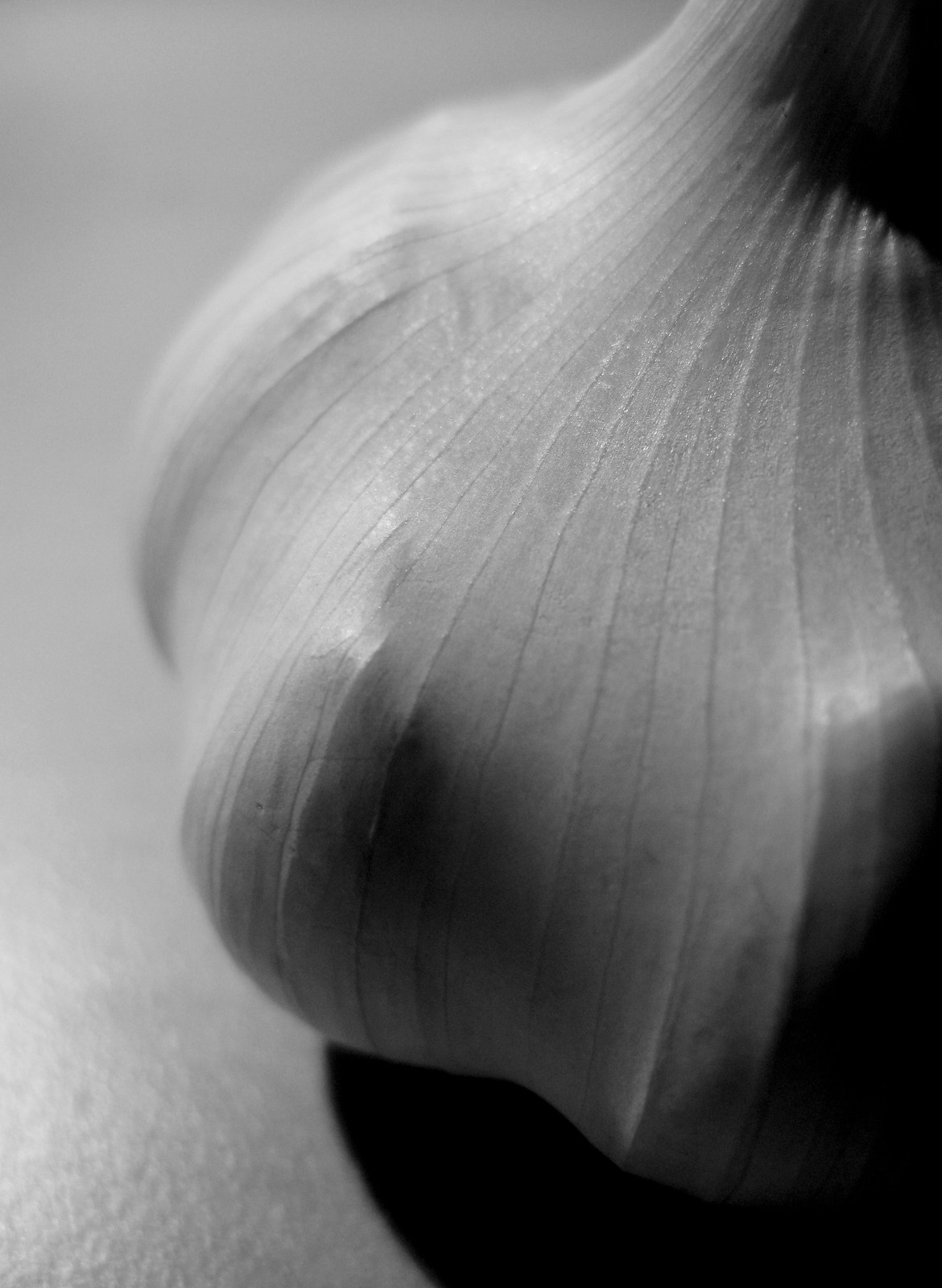This is a striking, black and white macro photograph of a whole garlic bulb, not individual cloves. The image captures the garlic in exquisite detail, focusing on the intricate lines and veins across its outer peel. The garlic, standing upright on a flat, light-colored surface that has a skin-like texture, is framed with its top right corner and part of the right side cut off. The left side of the image fades into a blurred white and gray background, while the bottom right shows a pronounced black shadow extending from the bulb. The curved edges of the individual cloves push against the skin, creating a textured, almost three-dimensional effect that emphasizes the natural beauty of the garlic. The portrait orientation of the image adds to its artistic flair, providing a close, crisp, and clear depiction of this everyday object.